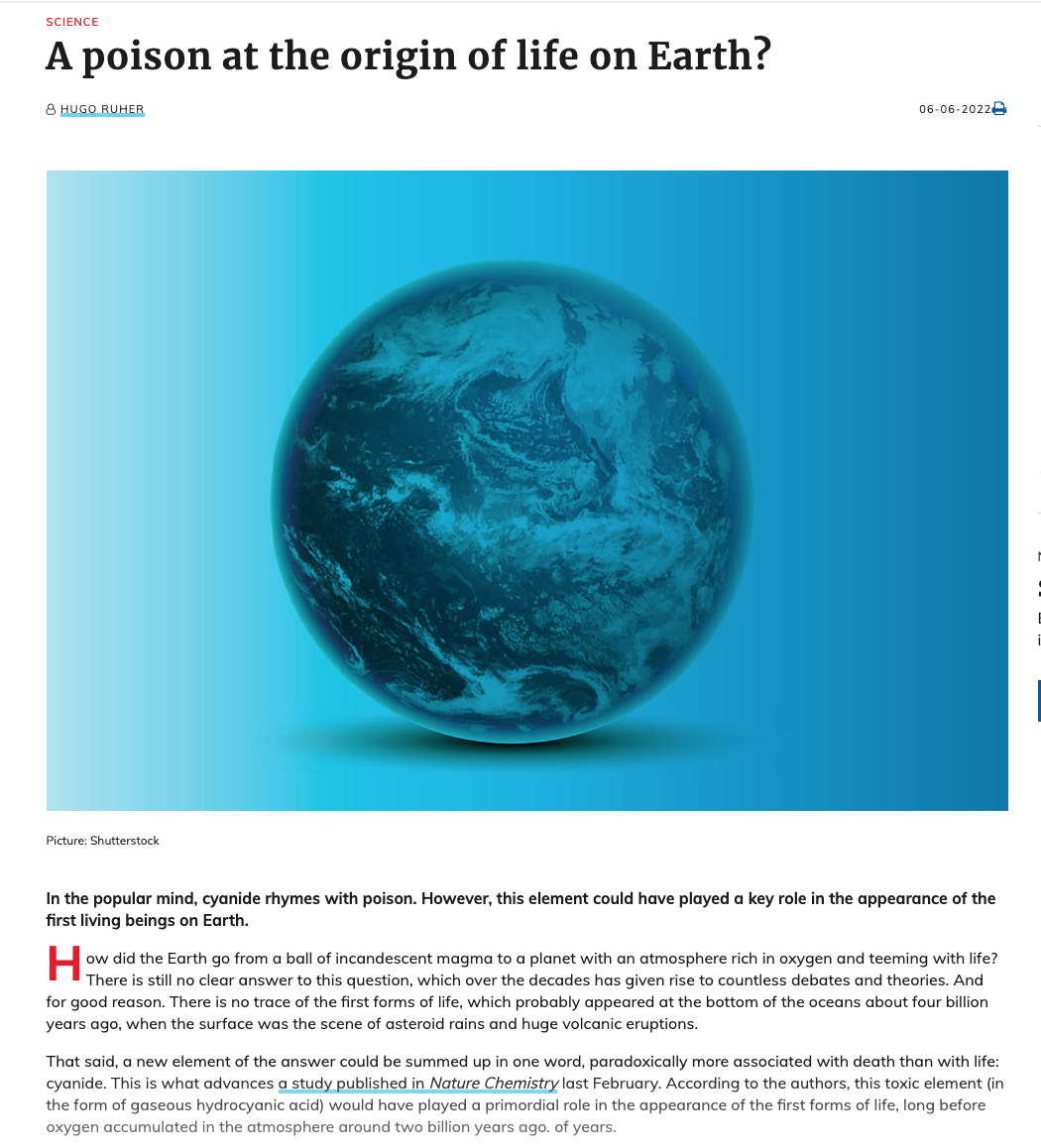**Science Article on Cyanide's Role in Early Life Formations**

*Science* - in small red font

**A Poison at the Origin of Life on Earth**  
*by Hugo Rueher*  
*Published on June 6, 2022* 

*[Print Article]*

*Image Credit: Shutterstock*

---

In the popular mind, cyanide rhymes with poison. However, this element could have played a key role in the appearance of the first living beings on Earth. The article explores how Earth transitioned from a ball of incandescent magma to a planet with an oxygen-rich atmosphere teeming with life. The origin of the first life forms remains a mystery due to the lack of traceable evidence, which probably appeared at the ocean floors about 4 billion years ago amidst asteroid rains and extensive volcanic eruptions. 

A potentially groundbreaking study published in *Nature Chemistry* last February argues that cyanide, specifically in the form of gaseous hydrocyanic acid, may have been crucial in the emergence of early life, predating the accumulation of atmospheric oxygen by approximately 2 billion years.